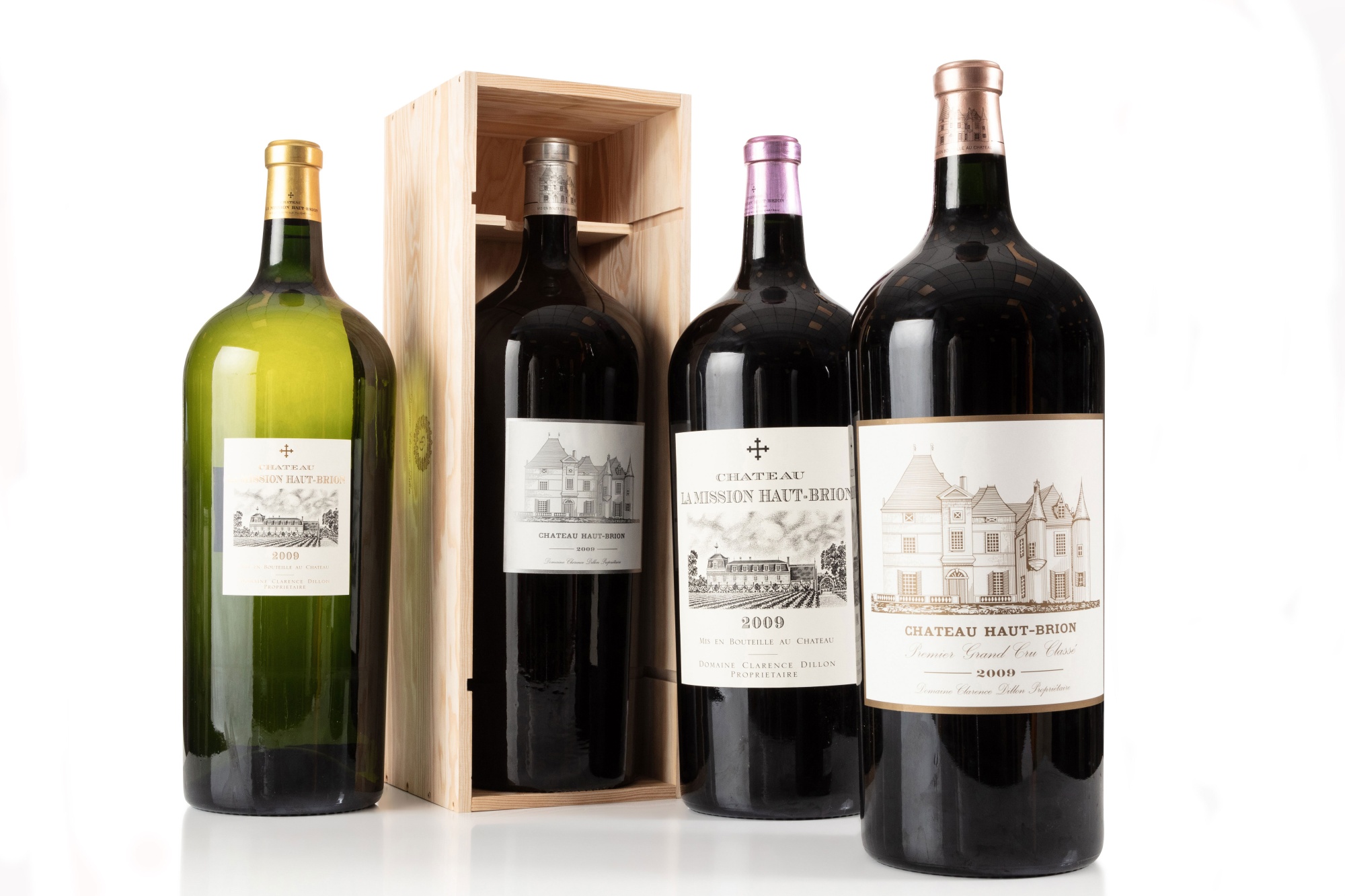The image is a photograph featuring four wine bottles displayed on a white surface, mimicking a wine catalog presentation. Starting from the left, the first bottle is a greenish-tinted bottle of white wine. It bears a white label with a hand-drawn black-and-white illustration of a vineyard, complete with a building in the background. 

Moving right, the second bottle is housed within a wooden case and is a dark bottle of red wine. It has a white label depicting an old-fashioned house or mansion in black and white, with a date and additional text.

The third bottle, also red wine, sits partially obstructed by the bottle to its right. It features a white label with an illustration similar to the leftmost bottle's vineyard image and a date of 2009 below the picture.

The fourth and closest bottle to the right is a dark bottle of red wine capped with gold foil. Its white label reads "Chateau Haut-Brion" above a black-and-white illustration of a building. This bottle also bears the year 2009 and more small writing beneath the illustration, creating a cohesive theme among these prestigious bottles of wine.